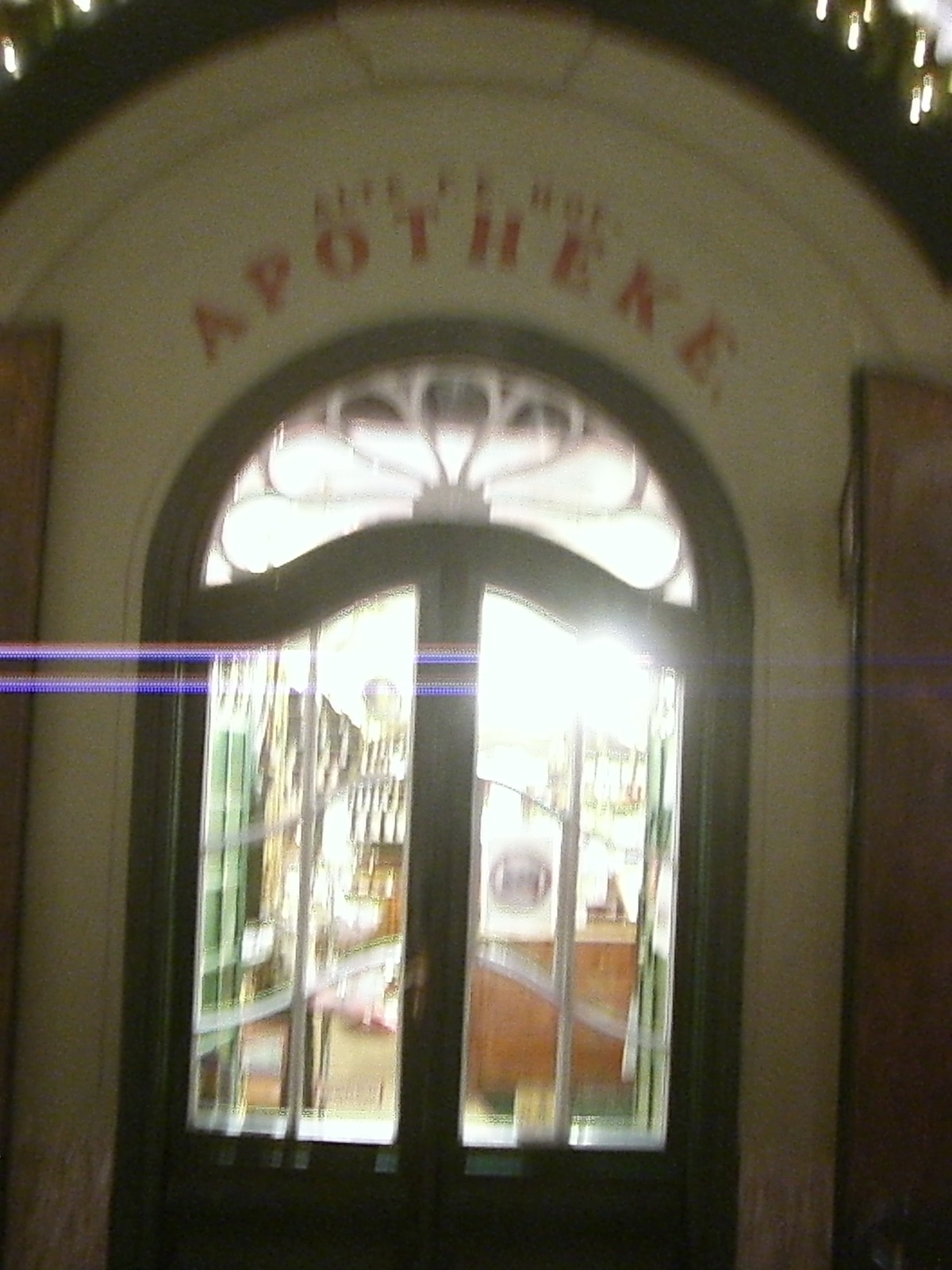This is a blurry photograph of the entrance of a building that appears to be a church or perhaps an apothecary store. The beige stone entrance features red text, possibly reading "life of Apotheke," above a wooden doorway with glass panes that allow a clear view inside. The doorway, with its cross-like design, has a vintage architectural style, including a semicircular arch with a patterned half-moon-shaped glass window at the top. Inside, the room is brightly lit despite it being night outside, revealing a variety of items on shelves and desks, resembling a store setup. The glass reflects light, casting two blue lines horizontally across the image. The entrance also includes vertical wooden panels on either side, adding to the classic and somewhat ambiguous nature of this building's purpose.